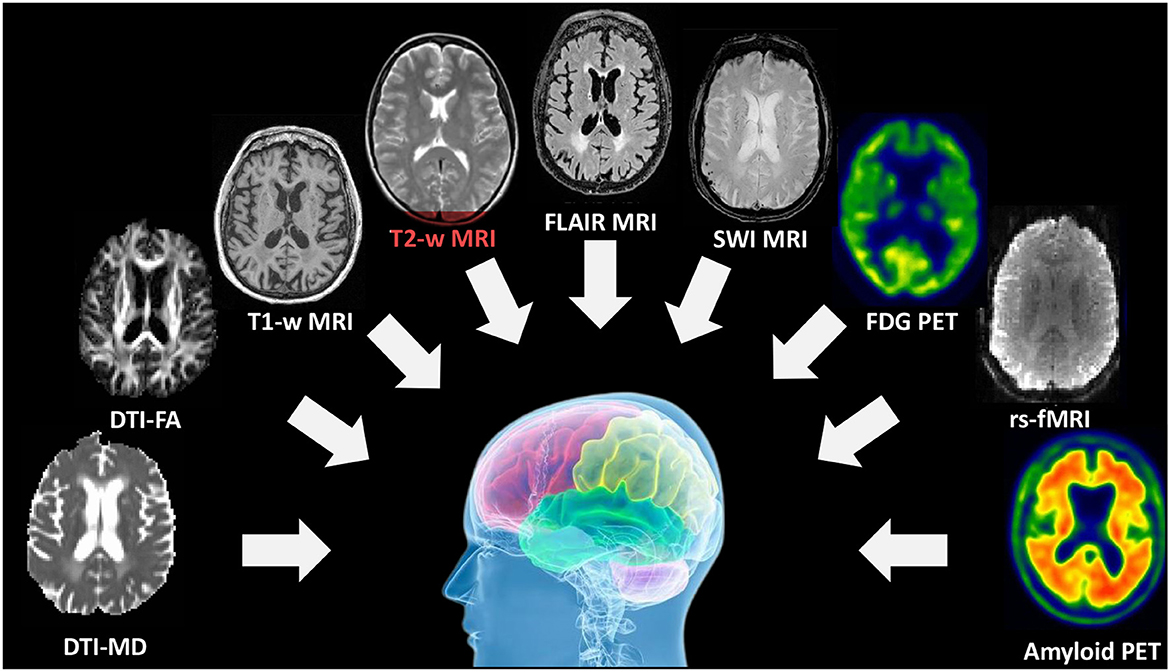The image displays a detailed visualization of brain scans, both in radiographic and color illustration formats, arranged within a rectangular frame where the top and bottom are twice as long as the left and right sides. At its center is a semi-transparent, light blue profile illustration of a human head, revealing a vibrant, color-coded representation of various brain sections in teal, yellow, and pink hues, with the spine faintly visible behind. The head is encircled by an arc of nine distinct brain scan slices, labeled beneath with scientific notation, marked as DTI-MD, DTI-FA, T1-WMRI, T2-WMRI, FLARE-MRI, SWI-MRI, FDG-PET, RS-FMRI, and AMYLOID-PET, starting from the bottom left and moving clockwise. Each scan slice features a corresponding white arrow pointing towards the central head, effectively linking each type of scan to its respective brain region. The entire composition is set against a stark black background, emphasizing the bright, neon colors and detailed anatomy, creating a vivid, graphically designed layout that blends radiographic imagery with illustrative elements.